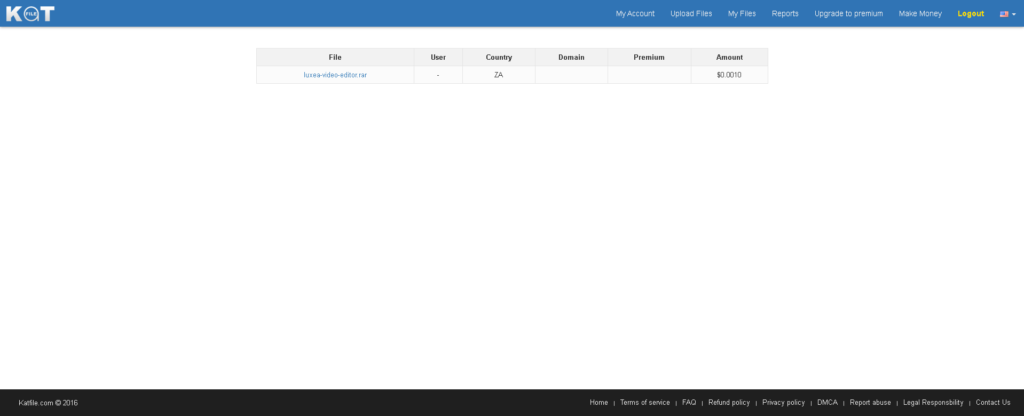The image displays the back-end of a user's account on an unspecified website, possibly a cloud file hosting service, judging by the layout and functionalities available. At the very top, there's a blue header bar featuring the website's logo in the far left corner. The menu bar, reading from left to right, includes the options: My Account, Upload Files, My Files, Reports, Upgrade to Premium, Make Money, and Logout.

Below the header, the main portion of the screen is mostly white and nearly empty, except for a small, fuzzy table. The table contains the headings: File, Country, Domain, Premium, and Amount. A hyperlinked file is listed under the File column, hinting at the presence of at least one uploaded file in this account. Due to the lack of additional context and clarity, the precise nature of this website remains unclear, although it suggests capabilities related to file management and possibly monetization features.